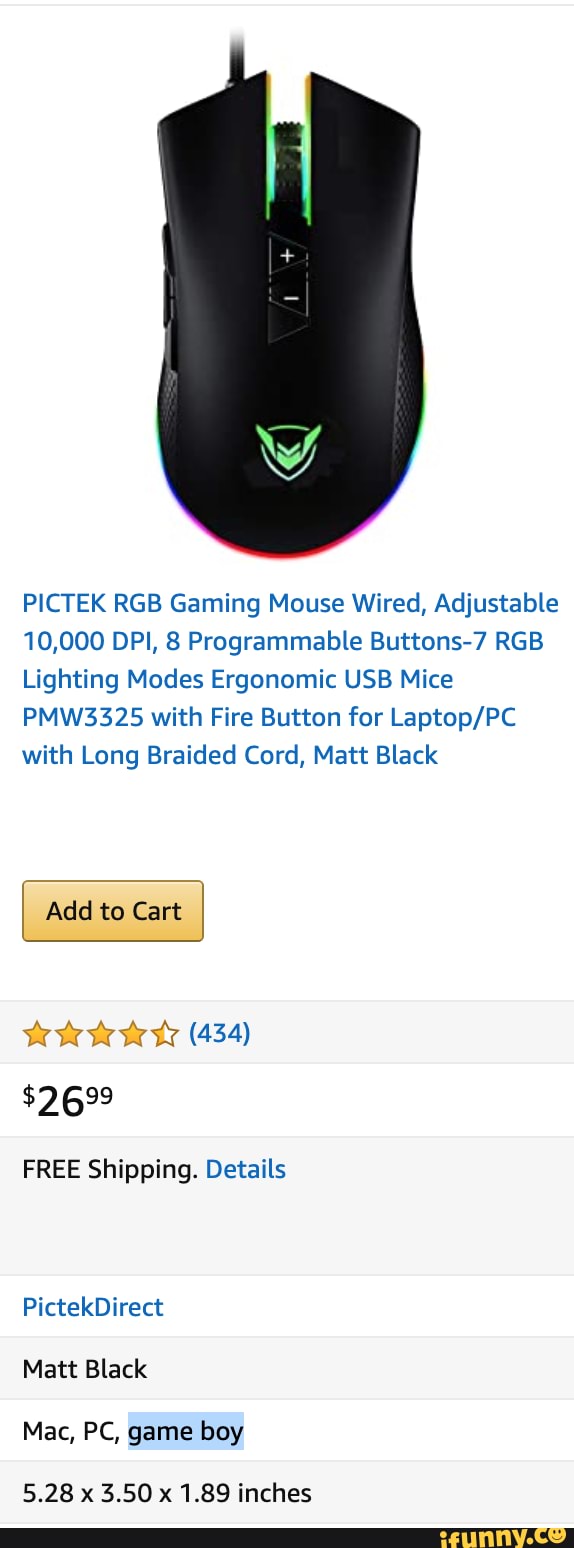The photo, captured from someone's cell phone screen, displays a detailed view of a gaming mouse product page. The focal point of the image is a sleek, matte black, wired gaming mouse prominently lit with a greenish-teal hue in specific areas. The mouse features a distinctive design with square edges near the top that smoothly transition into a curved bottom, and it bears a boomerang emblem at its base. A clear, visible cord extends from the top of the device, indicating its wired nature.

Below the image of the mouse, the text reads "PICTECH RGB Gaming Mouse, Wired, Adjustable, 10,000 DPI, Eight Programmable Buttons, Seven RGB Lighting Modes, Ergonomic, USB Mouse." Additional details mention that the mouse includes a "fire button" and comes with a long braided cord, all for a price of $26.99. With a rating of four and a half stars from 434 reviews, the listing also highlights free shipping. A conspicuous "Add to Cart" button is present, inviting users to make a purchase.